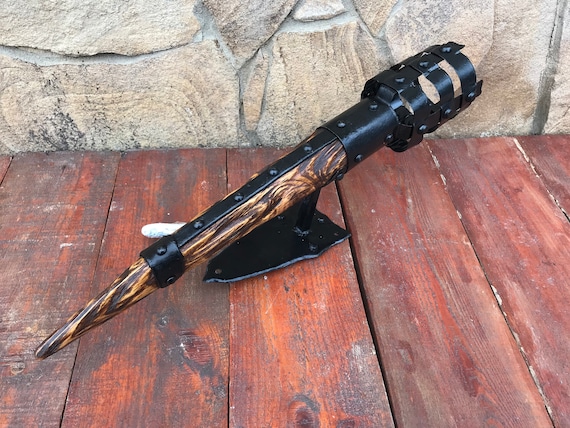The image features a detailed scene centered around a unique, carved wooden object on a reddish-brown wooden table. The object resembles a long, defied piece of wood with a marbled appearance, combining light and dark brown shades with a shiny finish. One end of the wood is pointed, while the other is rounded. Encircling the central wooden piece is a black metal sleeve, adorned with rivets, which appears to be securely attached. This sleeve tapers from a wider top section to a narrower one around the wood. The entire structure is mounted on a black metal stand, giving it a stable base. The background reveals a stone wall, adding a rustic ambiance to the setting.